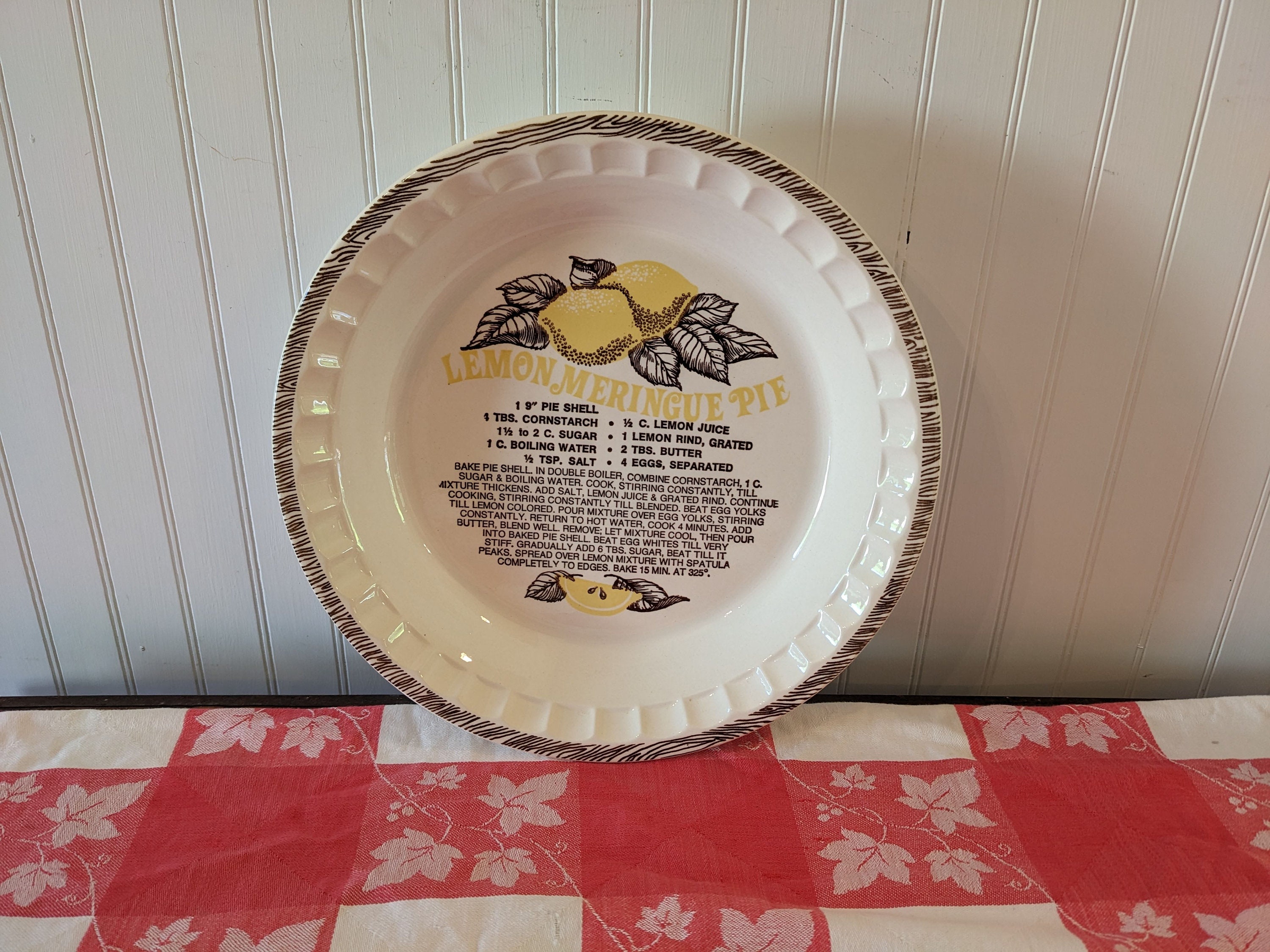The photograph, taken indoors, showcases a scene centered around a white wooden wall comprised of thin vertical slats with beveled edges. Below this wall sits a table or counter adorned with a red and white checkered tablecloth, which has white leaf prints decorating some of the red squares. This tablecloth appears to be made of plastic. Leaning against the wall is a large circular ceramic pie plate. The plate is predominantly white with black sketch-style decorations around its rim. The center of the plate features a vivid illustration of two lemons flanked by black leaves, as well as a lemon slice with leaves beneath it. In bold yellow text, the plate reads "Lemon Meringue Pie." Beneath this title, detailed in black text, is a comprehensive list of ingredients, such as salt, eggs, and lemon rinds. Further down, additional smaller black text provides step-by-step directions, instructing on preparation methods like cooking for four minutes and mixing the ingredients well.